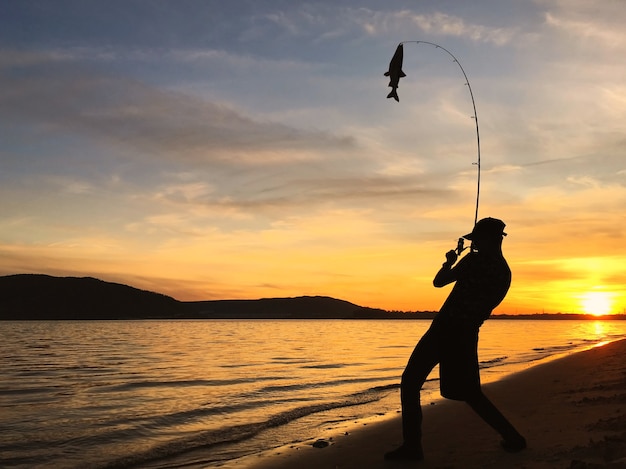In this photograph, taken at sunset, a man is silhouetted while fishing against a breathtaking, golden-hued sky. The sun sets to the right, casting a radiant glow across the tranquil water, which stretches out, reflecting the vibrant yellow and orange tones of the sky. The silhouette of the fisherman stands out on the right side of the image, his figure entirely in shadow as he holds a fishing pole high above his head, with a freshly caught fish dangling from the line. He appears to be wearing a baseball cap and possibly has a sack draped over his shoulder as he balances with bent knees on the sandy shore. To the left, the shadows of mountains frame the serene scene, bathed in the warm hues of the setting sun amidst a sky dotted with clouds. The overall composition captures a peaceful moment of triumph and natural beauty.